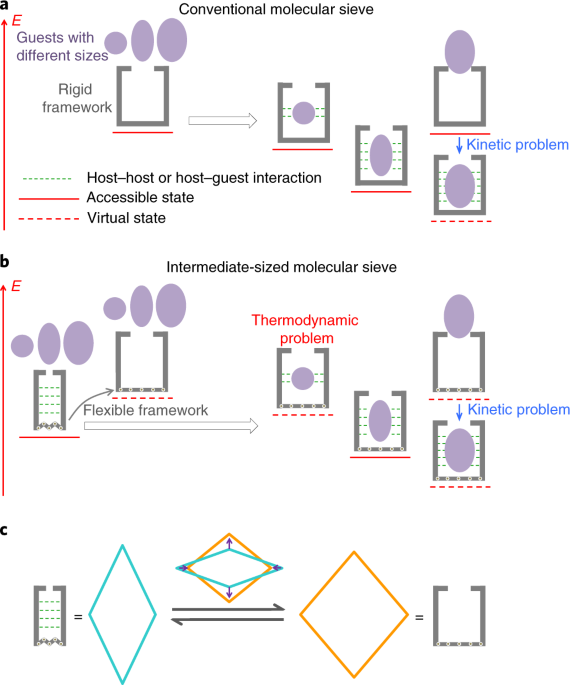This scientific diagram on a white background comprises three sections labeled A, B, and C, stacked vertically in a poster format. 

**Section A**, titled "Conventional Molecular Sieve" in black, features a series of diagrams illustrating "guests with different sizes." It depicts squares (representing a rigid framework) containing various shapes: purple circles and ovals. Some squares illustrate kinetic problems where the shapes cannot fit into the squares, labeled with dashed dotted lines indicating host-host or host-guest interaction, solid red lines for accessible states, and red dashed lines for virtual states. 

**Section B**, labeled "Intermediate Size Molecular Sieve," follows a similar pattern to Section A but focuses on a flexible framework. It also highlights thermodynamic and kinetic problems, with diagrams showing black squares and purple shapes experiencing similar issues due to size incompatibility.

**Section C** lacks a title and is populated with an array of colorful shapes including blue triangles, yellow tilted squares, and gray boxes, demonstrating some form of molecular interaction without specific annotations.

Overall, the diagram uses a combination of colors (purple, red, blue, yellow, gray) and lines to differentiate states and interactions, offering a detailed schematic representation of molecular sieves and their corresponding frameworks and issues.